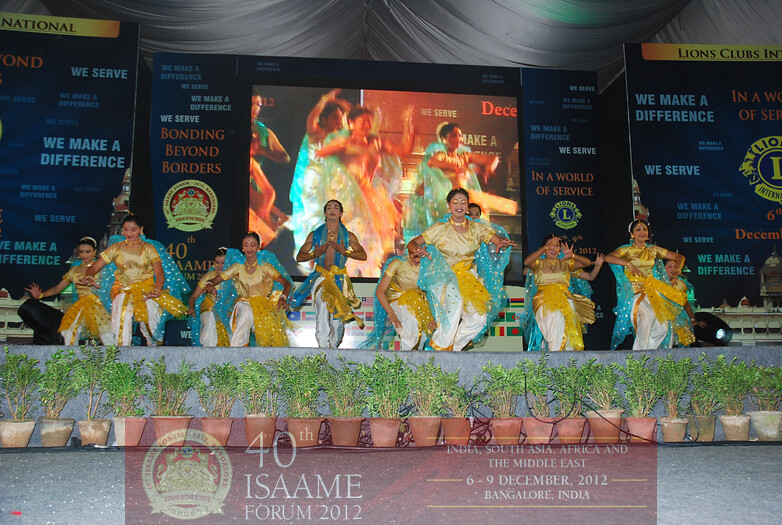The image captures a vibrant stage performance in Bangalore, India, taking place at the 40th ISAAME Forum held from December 6th to 9th, 2012. The outdoor stage is adorned with potted plants lining the front, and a graphic displays the event name. Approximately a dozen dancers, comprising mostly women but with some men, are energetically performing in traditional Indian clothing characterized by white pants, gold tops, and teal-colored scarves and sashes. The dancers' outfits are further accentuated with gold accessories, including bright gold sashes and makeup. Behind them, a large screen projects their dance, while the stage backdrop bears phrases such as "We serve," "We make a difference," "Bonding beyond borders," and "Lions Club International." The vivacious scene radiates cultural richness and unity, embodying the theme of international service and camaraderie.